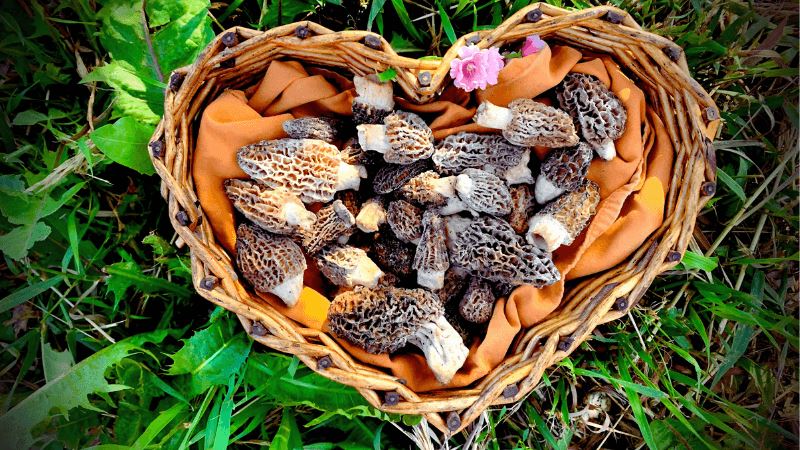A heart-shaped woven reed basket, light brown in color, sits on a lush bed of green grass, accompanied by a single dandelion. Inside the basket, an orange cloth cushions an abundant collection of morel mushrooms, known for their spongy, darkish brown to light brown conical caps and white, tapered stalks. Among the mushrooms, a delicate pink posy flower adds a touch of color. The vibrant, detailed scene appears almost too perfect, suggesting it might be computer-generated or an exceptionally vivid photograph. The image is taken from a top-down perspective, showcasing both the intricate design of the basket and the natural elements around it.